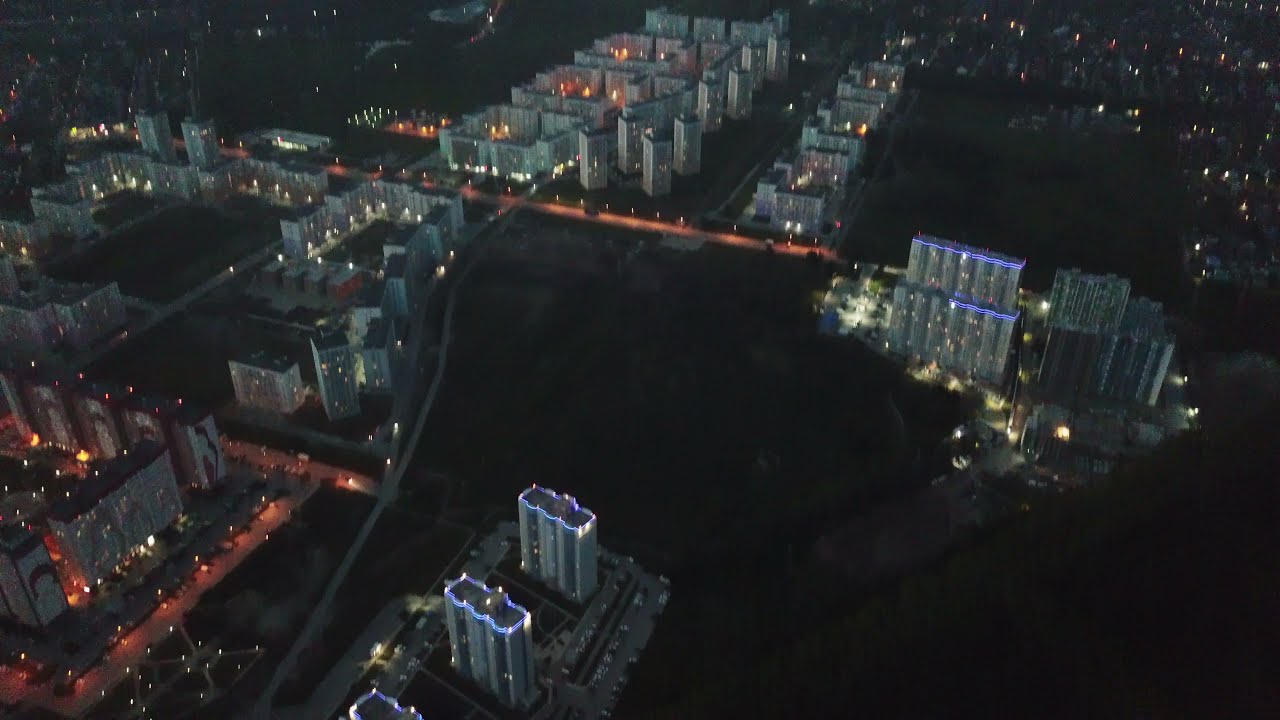The image is an aerial, nighttime color photograph of a cityscape, captured from several hundred feet above, possibly by a drone. The landscape orientation reveals a dimly lit urban environment, dominated by numerous high-rise, commercial buildings. The buildings, predominantly gray and light-colored, are regularly aligned and vary in shape—some are thin and rectangular, others wide and rectangular, while some are shorter and more square. These structures are organized in a grid pattern, with streets meeting mostly perpendicularly.

In the forefront and throughout the photograph, the buildings are densely packed, particularly in the downtown area. However, the image also features significant dark patches, likely indicating areas of vegetation or undeveloped lots.

Prominent in the photo are three rectangular buildings in the foreground, two fully visible and one partially so. The buildings are illuminated by light emanating from their windows and from lights on their rooftops. An island-shaped area on the right side of the image boasts additional high-rise buildings and scattered lights, with the upper right corner showing a cluster of more residential-looking homes, their presence marked by several glowing windows.

At the bottom left corner, a rectangular building complex is distinguished by orange-colored lighting on the ground. The scene’s composition, combined with the subdued nighttime ambiance, reflects a style of photographic representationalism and realism.